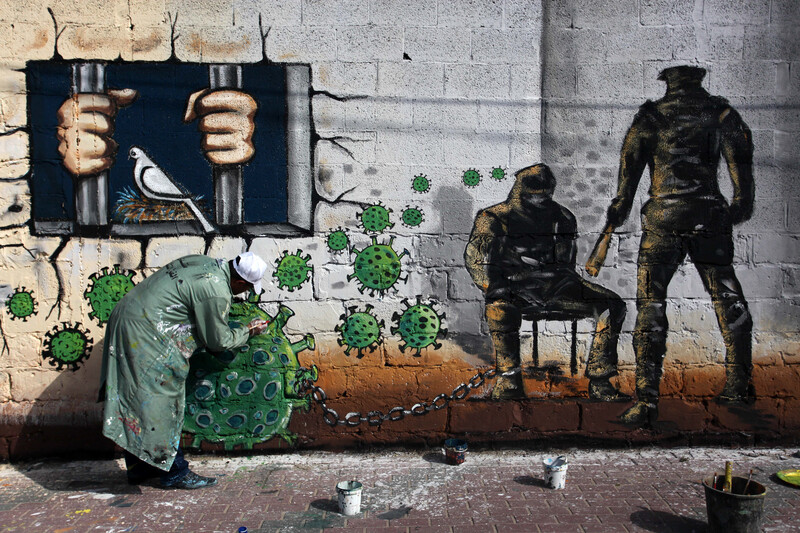In this vibrant and detailed mural set against a brick wall and flooring, an artist in a green coat spattered with paint, black paint-covered shoes, and a white hat is seen crouched to the left, engrossed in painting. With a paintbrush in hand, the artist meticulously works on what seems to be a large COVID-shaped virus encircled by smaller virus drawings, enveloped in smoke. To the left of the mural is a striking scene of two hands gripping prison bars, peering out from a cell window. Centrally, a bird perches on a colorful nest, a symbol of fragility amidst chaos. To the right, the mural takes a darker turn, depicting a hostage bound to a chair with an ankle chain linking him to the virus the artist is painting. The hostage, with their face covered and head bowed, is menaced by a man in battle camouflage holding a glass bottle, creating a tense, thrilling atmosphere. Paint buckets and brushes are scattered across the brick floor, capturing the ongoing artistic endeavor that interweaves themes of confinement, disease, and conflict in a powerful political message.